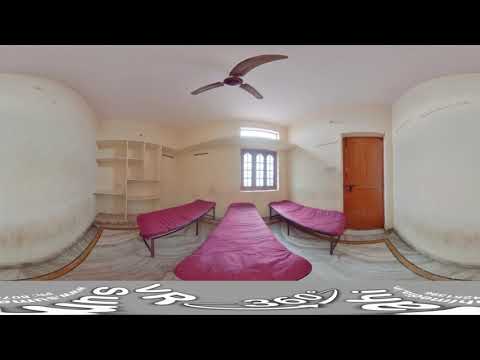This fisheye lens image captures the interior of what appears to be a massage studio or similar setting. The composition is defined by a solid black border at the top and bottom, with a gray banner just above the bottom edge displaying "VR 360." Central to the image are three beds with purple coverings, arranged around a window that allows light to stream in, hinting at a midday timeframe. The surrounding walls are a soft beige or off-white color, with various other colors visible in the scene including tan, gray, pink, and purple. In the upper portion of the image, a ceiling fan is present, its blades appearing curved due to the fisheye effect. A brown or reddish-brown door is visible on the right side, near the beds. The floor has a smooth, grayish appearance with a perimeter stripe. On the left side, empty shelving units can be seen. The entire setting gives off a tranquil, organized ambiance suitable for a place designed for relaxation.